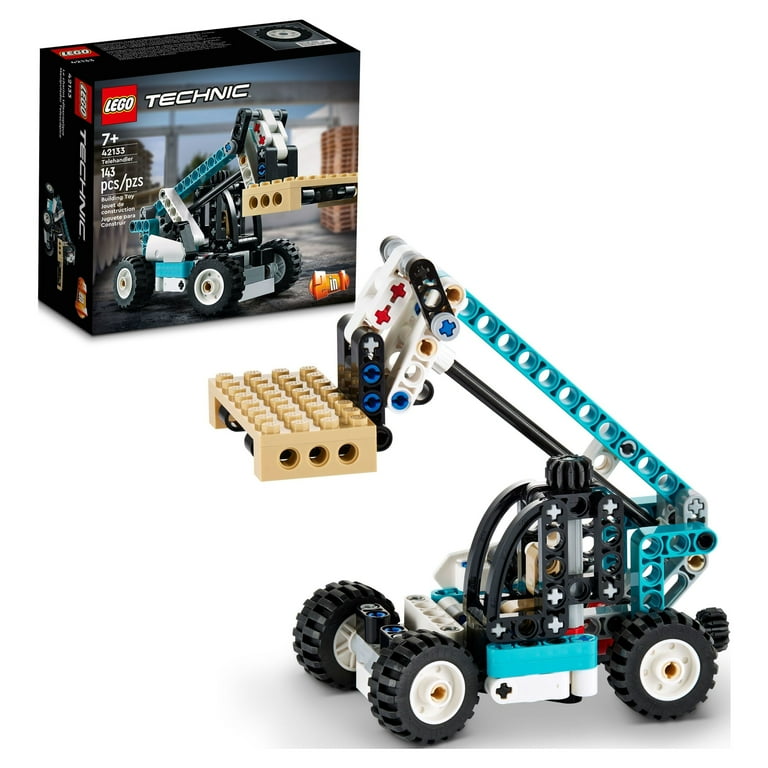A color photo on a white background showcases the LEGO Technic kit 42153, designated for ages H7+, with 143 pieces. Prominently displayed in the top left is the box, which features a red LEGO logo, an image of the completed model, and the "LEGO Technic" branding, all set against a predominantly black background. The box also notes in large orange letters that the kit offers a "2-in-1" build option. To the right, the completed LEGO model is presented—a robust, crane-like forklift with four large, off-road wheels. The main body of the vehicle is a blend of light blue and white, while the crane arm extending from the base is a striking turquoise. The arm attaches to a tan, almost light yellowish-brown platform, with a black rod providing additional support. The crane is designed to lift pallets, with visible red, blue, and grey pins connecting the various components, exemplifying the detailed construction typical of LEGO Technic sets.